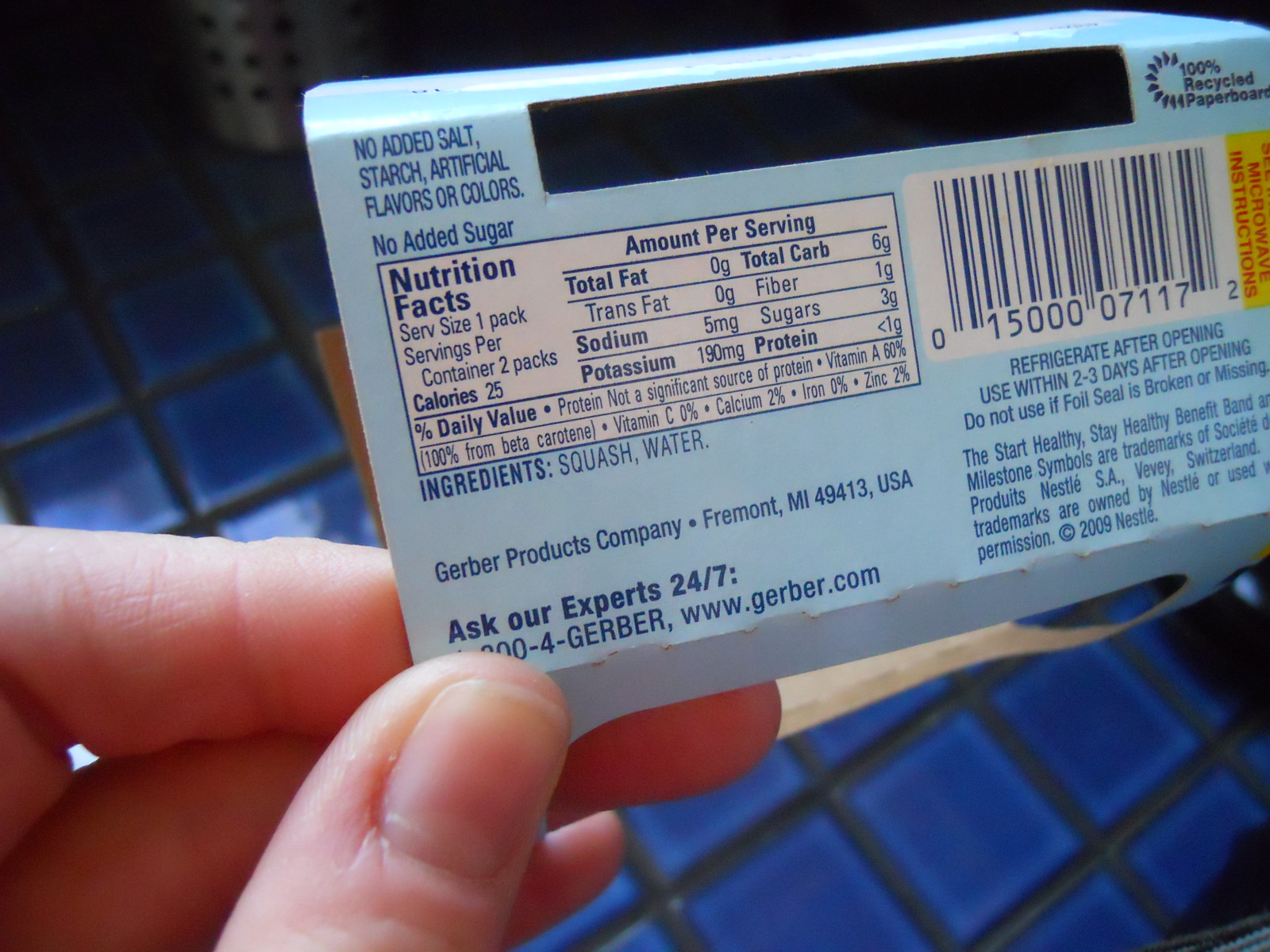This first-person POV close-up image captures the back of a cardboard package, focusing on the nutritional label and barcode. The nutritional table is prominently displayed on the left-hand side, detailing:

- Serving Size: 1 pack
- Servings Per Container: 2 packs
- Calories: 25 per serving
- Total Fat: 0 grams
- Trans Fat: 0 grams
- Sodium: 5 milligrams
- Potassium: 190 milligrams
- Total Carbohydrates: 6 grams
  - Sugars: 3 grams
  - Dietary Fiber: 1 gram
- Protein: Less than 1 gram (Note: Not a significant source of protein)
- Vitamin A: 60% (100% from beta-carotene)
- Vitamin C: 0%
- Calcium: 2%
- Iron: 0%
- Zinc: 2%

To the right of the nutritional facts is the barcode. Below the barcode are instructions that state: "Refrigerate after opening. Use within two to three days after opening. Do not use if foil seal is broken or missing."

The nutritional details and instructions are all set against a blue-colored background on the cardboard packaging, providing clear and essential information for the consumer.